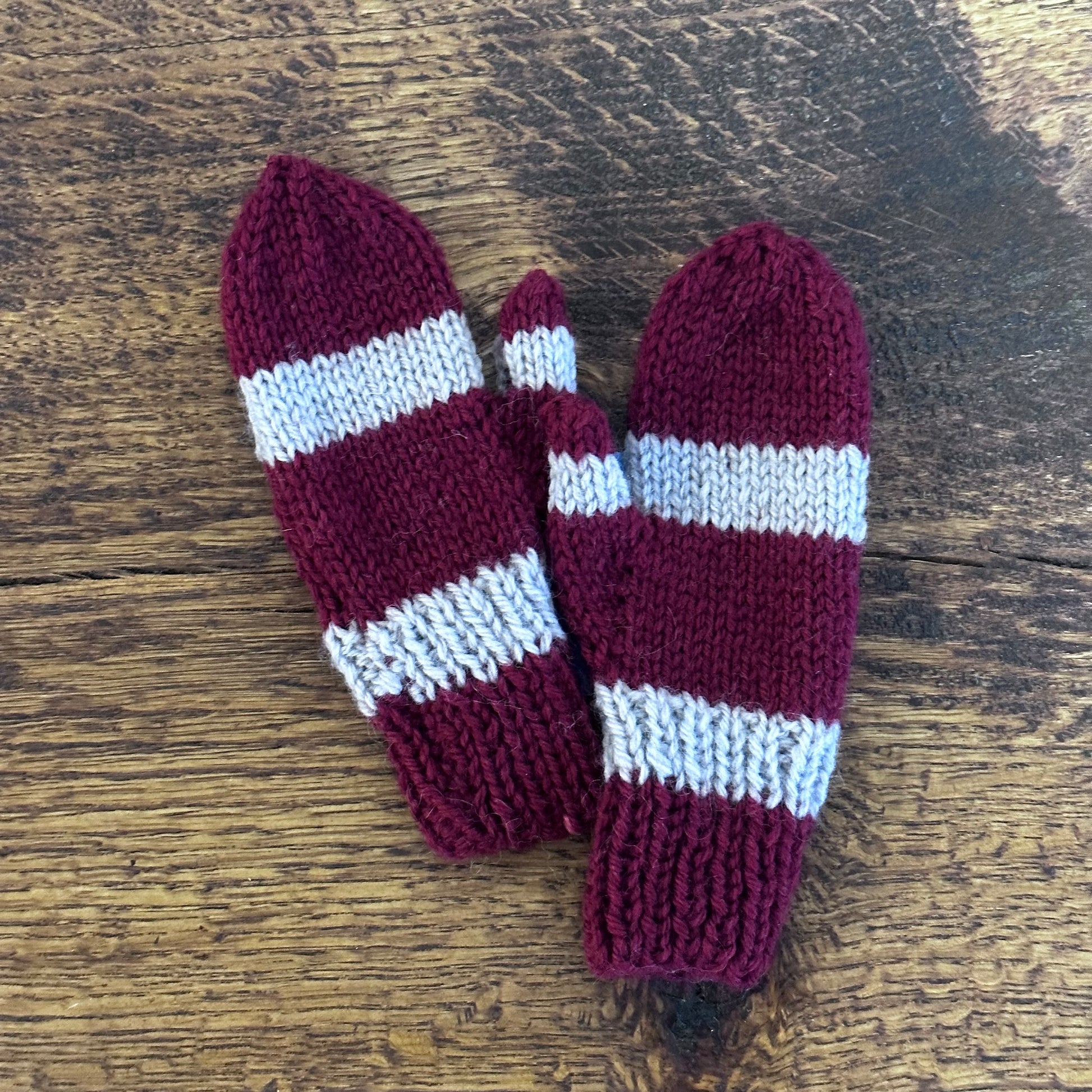In this vivid photograph, a pair of hand-knitted mittens is meticulously laid upon a rustic, aged brown wooden table. The table features a rough sawn texture, with blackened areas that add to its character. The mittens, which dominate the center of the image, boast a rich purplish magenta hue adorned with broad, light gray stripes. The stripes, carefully knitted to ensure consistency, run horizontally across each mitten—one stripe near the cuff and another positioned near the palm area. The mittens, showing hints of knitting inconsistencies, reveal two different knitting techniques: purl and regular knitting. The image highlights the artisanal quality of the mittens, suggesting they are designed for an adult. The bright, high-contrast nature of the photograph accentuates the vivid colors and textures, creating a striking depiction of these hand-crafted accessories.